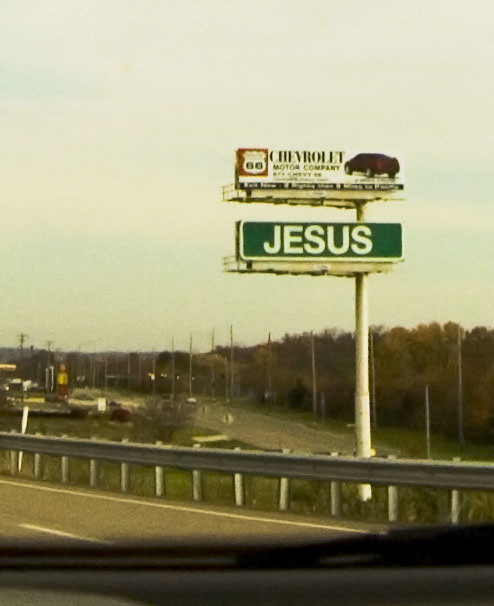The image captures a roadside view from inside a vehicle, with the edge of the dashboard and part of the window visible at the bottom of the frame. The asphalt road, marked with white painted lines, is flanked by a metal guardrail. The terrain appears to gently slope downward beyond the guardrail, revealing tall grass. Dominating the scene is a large white billboard supported by a substantial pole. The top portion of the billboard features an advertisement for the Chevrolet Motor Company, showcasing a red car against a backdrop of bold, clear graphics. Beneath this ad, a section of green background bears the word "Jesus" in capital white letters. The background of the image includes a distant road shaded by numerous trees. The sky above is predominantly white with soft hints of light blue breaking through.